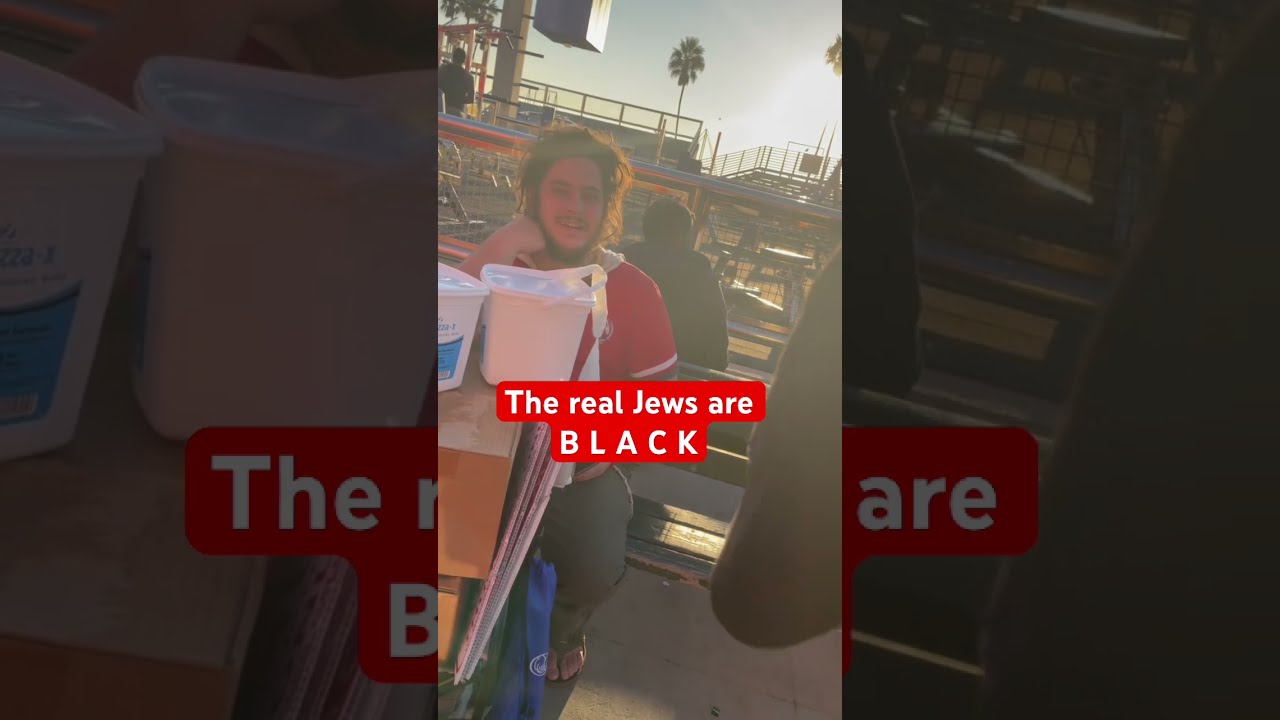In this image, a young man with frizzy, unkempt hair, a scraggly beard, and a thin mustache is seated at a table outdoors. He appears to be in his early 20s and is wearing a red t-shirt with a San Francisco 49ers logo and white and gold hems around the sleeves. Beneath the red shirt, a hoodie can be seen. The setting appears to be a public eating area near a beach, featuring palm trees, sandy patches, concrete, and picnic benches. On the table in front of him, there are a couple of white buckets and a trash can with a white handle. Other people and various buildings can be seen in the background, along with a clear sky, suggesting it's midday. The photo, likely a screenshot from a mobile app like TikTok or Instagram, prominently features white text on a red background in the center that states, "The real Jews are black." The color palette includes blue, brown, white, red, gray, green, and orange. The scene is likely part of a message or statement being shared by the subject.